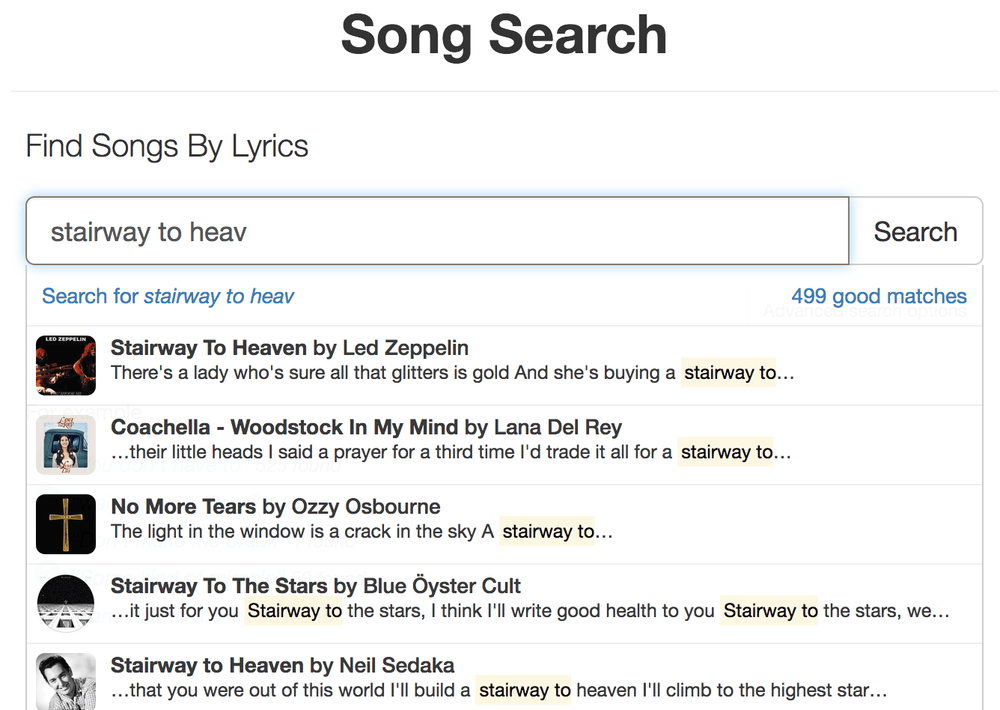The image is a screenshot of a web page specifically designed for song searches. The page features a white background with the heading "Song Search" prominently displayed in bold black letters at the top. Directly beneath the heading is a thin gray line extending horizontally across the page. Below this line, the words “Find songs by lyrics” are displayed, followed by a search bar. Inside the search bar, partially visible text reads "Stairway to Heaven," with the last part of "Heaven" cut off.

To the right of the search bar, a search button is visible. Below the search bar and search button, there is a line of blue text that reads, "Search for 'Stairway to Heaven'" and indicates "499 good matches" in blue.

The search results displayed include five different songs:

1. **"Stairway to Heaven" by Led Zeppelin**: This result includes an image of the band and displays the lyric snippet, "There's a lady who's sure all that glitters is gold, and she's buying a stairway to…"

2. **"Coachella, Woodstock in My Mind" by Lana Del Rey**: Accompanied by an album cover image, the lyric snippet shown is, "They're little heads, they said a prayer for a third time, I trade it all for a stairway to…"

3. **"No More Tears" by Ozzy Osbourne**: Featuring an image of a cross against a black background, the displayed lyrics include, "The light in the window is a crack in the sky, a stairway to…"

4. **"Stairway to the Stars" by Blue Öyster Cult**: The snippet reads, "It's just for you, Stairway to the Stars, I think I'll write good health to you. Stairway to the Stars, we…"

5. **"Stairway to Heaven" by Neil Sedaka**: This result includes the lyrics, "You are out of this world, I'll build a stairway to heaven, I'll climb to the highest star."

Each result is accompanied by an image relevant to the song or artist.